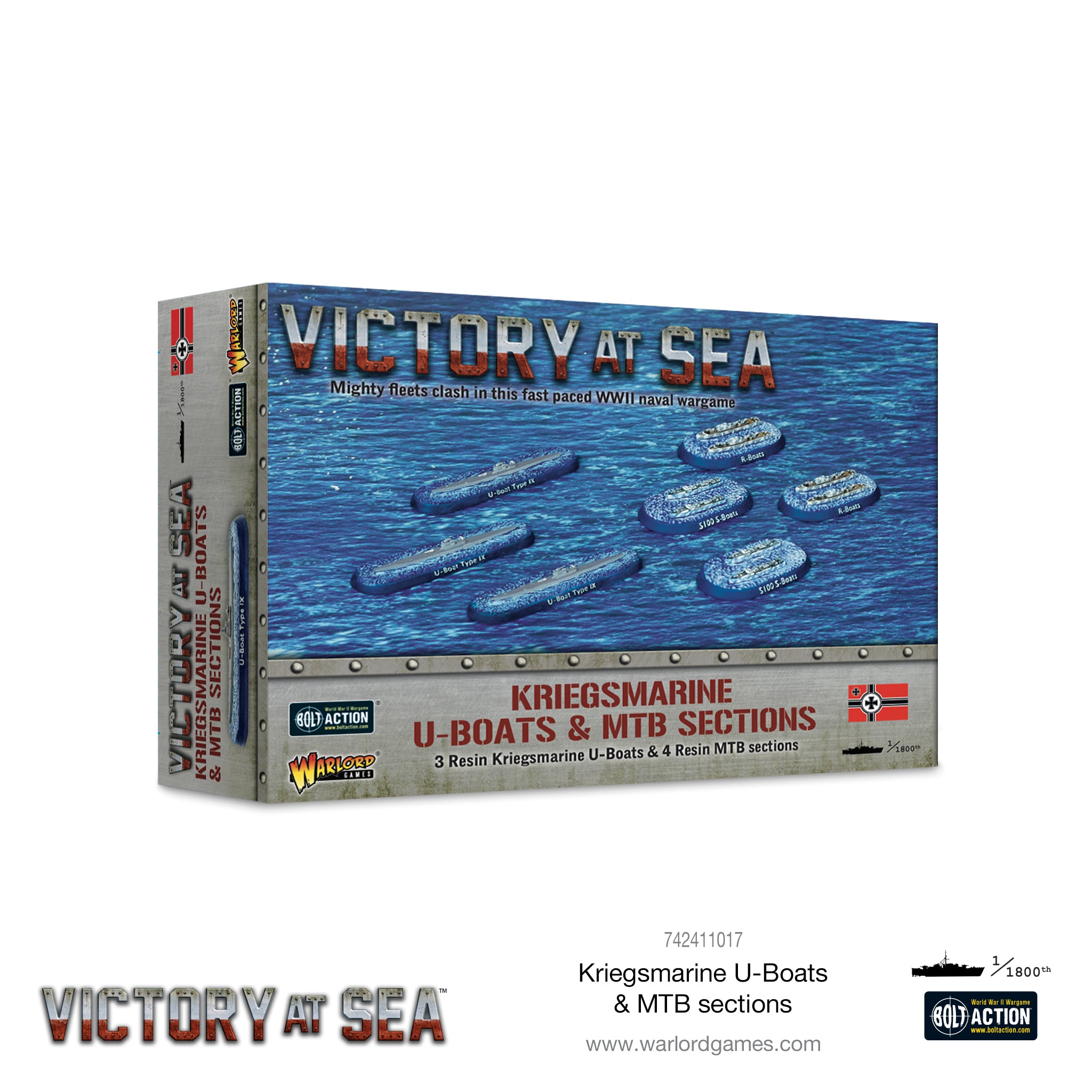This image depicts a vintage-looking box for a model set titled "Victory at Sea," featuring a World War II naval war game where mighty fleets clash in fast-paced battles. The box, primarily gray with a metal-like appearance and bolts illustrated, prominently displays the text "Victory at Sea" in red. The center showcases a blue-toned illustration of maritime action, including three resin Kriegsmarine U-boats resembling long pills and four smaller resin MTB sections shaped like smaller pills. The box also mentions, "Kriegsmarine U-boats and MTB sections," and indicates a scale of 1:1800, highlighting its detailed miniatures. The branding "Warlord" is visible, suggesting the manufacturer, with additional catalog information reading, "742-41017 Kriegsmarine U-boats and MTB sections."